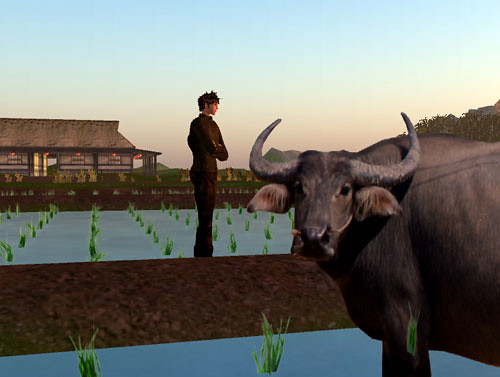The image appears to be a screenshot from a video game featuring CGI graphics with a surreal and low-resolution aesthetic. In the scene, a brown water buffalo stands in the foreground, turning its head to look directly at the viewer. It is situated near flooded plots containing organized rows of crops, resembling a rice paddy. In the middleground, a man with dark hair, wearing dark, brown attire, stands on the ground between the plots, arms crossed. The background reveals a farm setting with a one-story oriental-style building or house, characterized by its brown roof, white walls, and hanging lanterns. The sky above transitions from blue to a light violet-gray near the horizon.